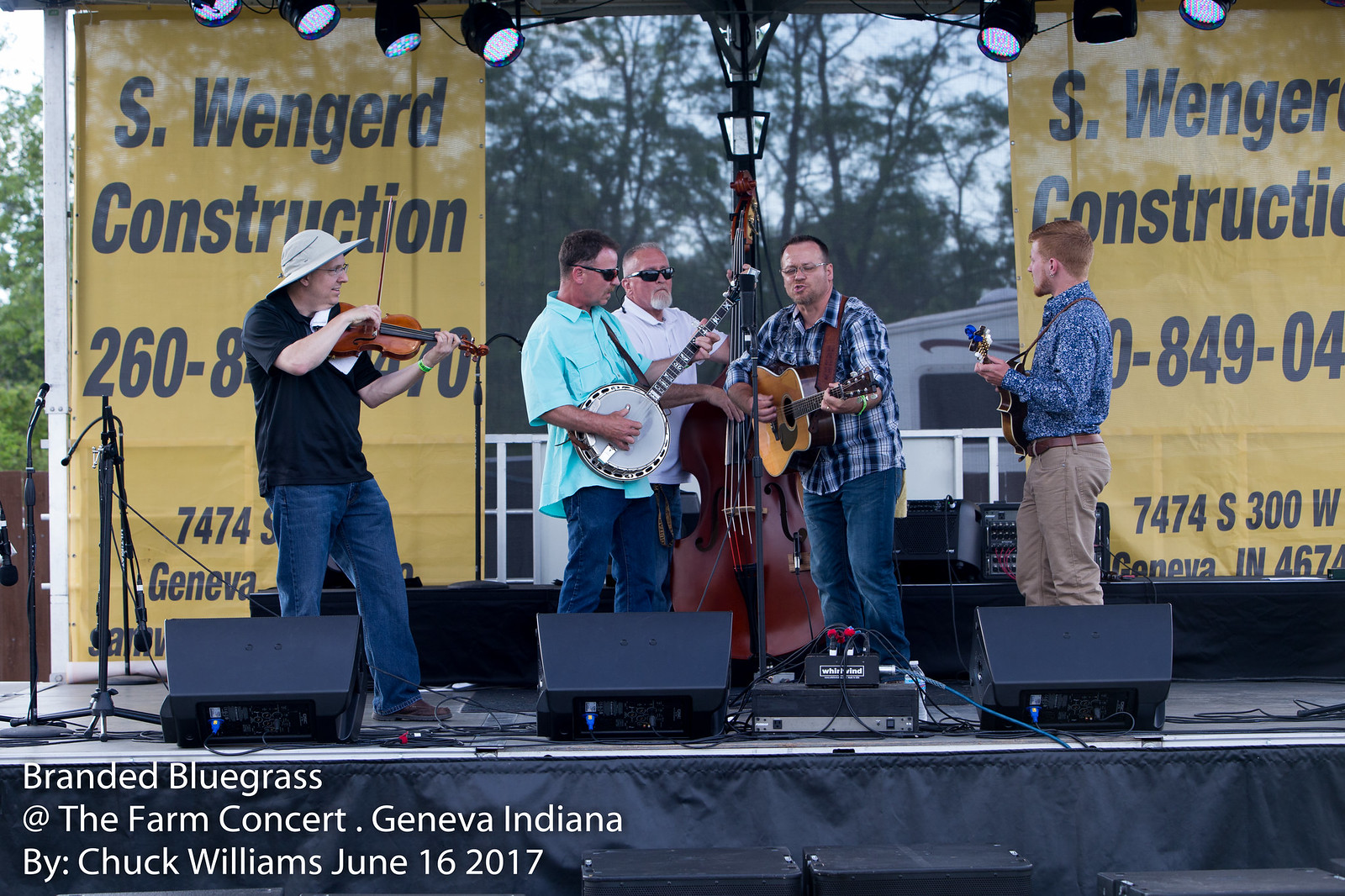This photograph, taken during the day at the Branded Bluegrass at the Farm Concert in Geneva, Indiana by Chuck Williams on June 16, 2017, showcases a lively outdoor performance on a well-equipped stage. Prominent at the bottom of the stage is white text on a gray background that reads "Branded Bluegrass at the Farm Concert, Geneva, Indiana by Chuck Williams, June 16, 2017." Flanking the stage sides are yellow banners from S. Wengard Construction, complete with phone numbers and addresses.

On stage, five musicians energetically play their instruments amidst an array of sound equipment, microphones, and lights. From left to right:
1. A violinist, distinguished by a white safari hat, black polo shirt, and blue jeans.
2. To his right, a banjo player in a light green shirt and blue jeans, sporting sunglasses.
3. Positioned centrally, a bassist in a white shirt, also wearing sunglasses, with his right hand on the upper strings of the bass.
4. A guitarist to the bassist's right, wearing a checkered blue and white shirt and blue jeans.
5. Finally, to the far right, a red-haired musician in a blue shirt and khaki pants, playing what appears to be another guitar.

The backdrop features a scenic mix of trees and a building, completing the setting for this down-to-earth musical event.